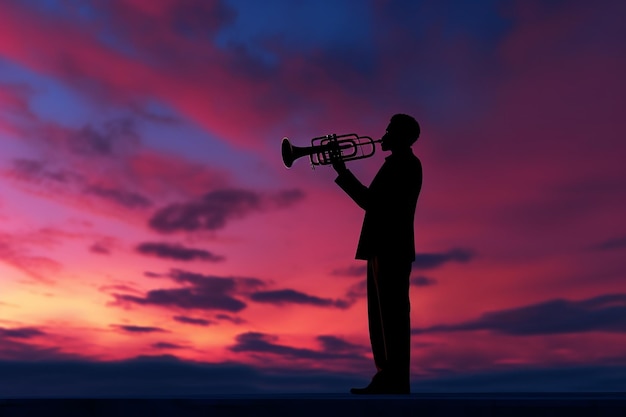A captivating silhouette of a jazz musician, dressed in a sport coat and pants, stands slightly off-center, playing a brass instrument that could be a flugelhorn, cornet, or modified trumpet. His profile is dark against the enchanting hues of a sunset or early sunrise sky, painted in shades of deep purple, pink, blue, and orange. The man's figure and instrument are silhouetted against wispy clouds and a thin, black horizon line. The sun, almost set, casts yellow highlights near the horizon, creating a striking contrast with the musician's silhouette. He stands on a flat surface, facing left, with the instrument raised to his lips, embodying the essence of jazz in this artistic and abstract photograph.